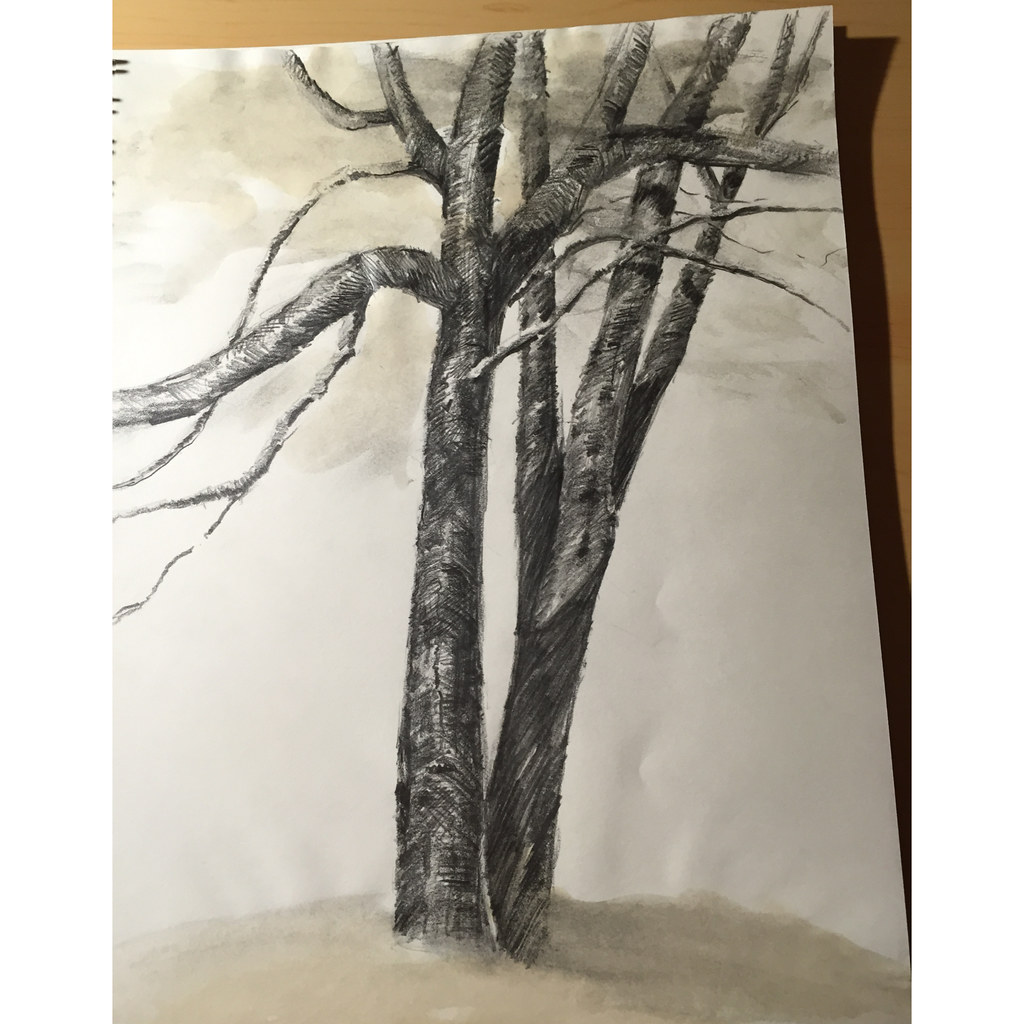This image features an intricately detailed drawing on a piece of paper. The artwork depicts two intertwined, bare trees prominently illustrated with charcoal, giving the branches a black, textured appearance with some highlights of light gray. The trees split about a foot above the ground, extending their numerous limbs in various directions. The ground beneath the trees is rendered in a light brown or beige color, resembling watercolor, and suggests a grassy but yellowish terrain. The background is a light orchid hue, adding a gentle contrast to the stark, bare branches. The backdrop is decorated with swirling light tan, possibly indicating clouds or an abstract representation of distant elements, though it doesn't resemble leaves. The drawing is meticulously shaded and presented against a brown desk or wall, accentuating its artistic quality and attention to detail.